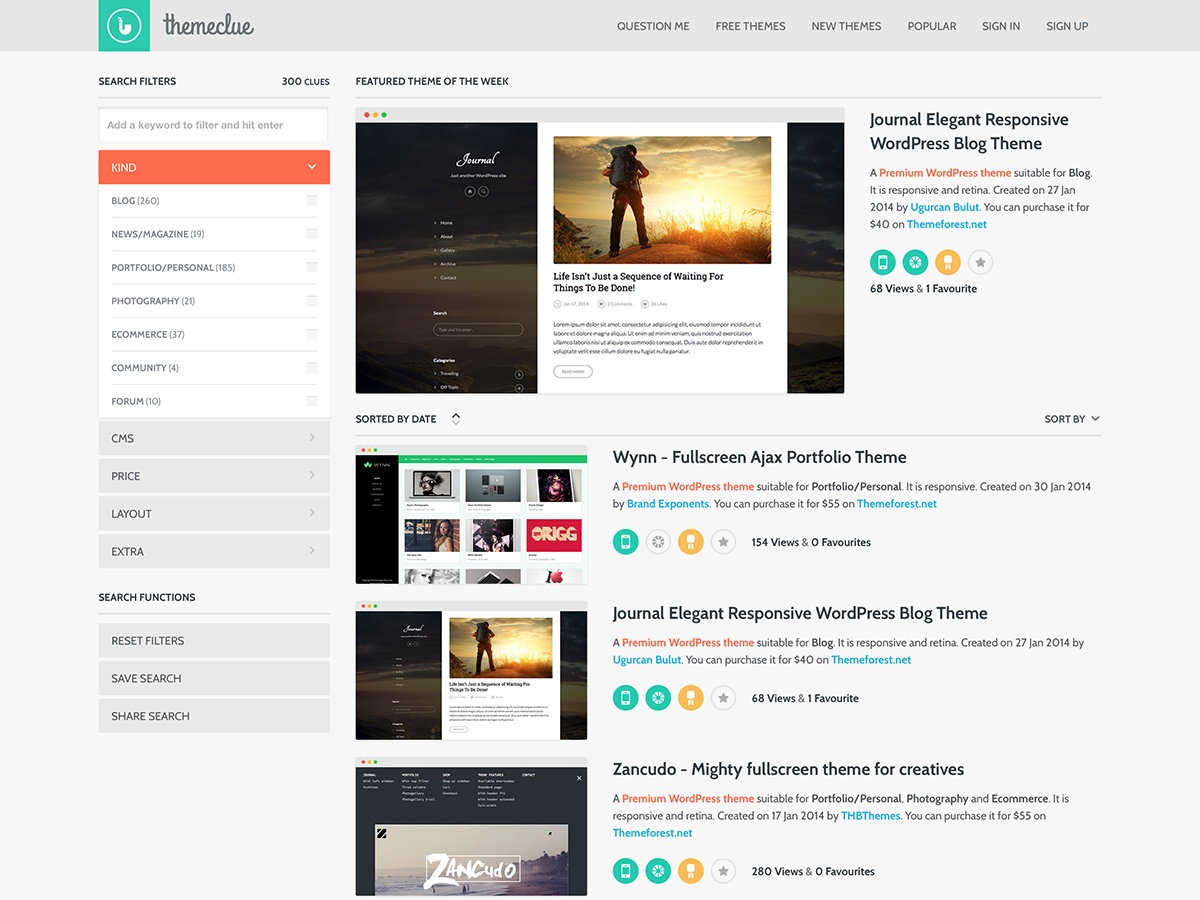This image captures a webpage displayed on a computer screen. At the top of the page, there is a title written in cursive black print that reads "Theme Clue." Beside the title, on the left, there is an icon of an old-fashioned smoking pipe with a curved design. Just below the title bar, there is a navigation menu with clickable options labeled "Question Me," "Free Themes," "New Themes," "Popular," "Sign In," and "Sign Up."

On the left side of the page, there's a sidebar labeled "Search Filters." It indicates that there are 300 clues available and provides an input box for users to add a keyword to filter these clues, with instructions to hit enter after typing. A highlighted keyword, "Kind," in an orangish-red color, is visible within the box. 

Below the search filter, several categories are listed, including "Blog," "News Magazine," "Portfolio Personal," "Photography," "E-commerce," "Community," and "Forum."

Centered on the page, there is a featured section titled "Featured Theme of the Week." In this section, a quote is displayed: "Life isn't just a sequence of waiting for things to be done." There is an option to click and read more about this feature. Just below, it describes the featured theme as a "Journal, Elegant, Responsive, WordPress Blog Theme."